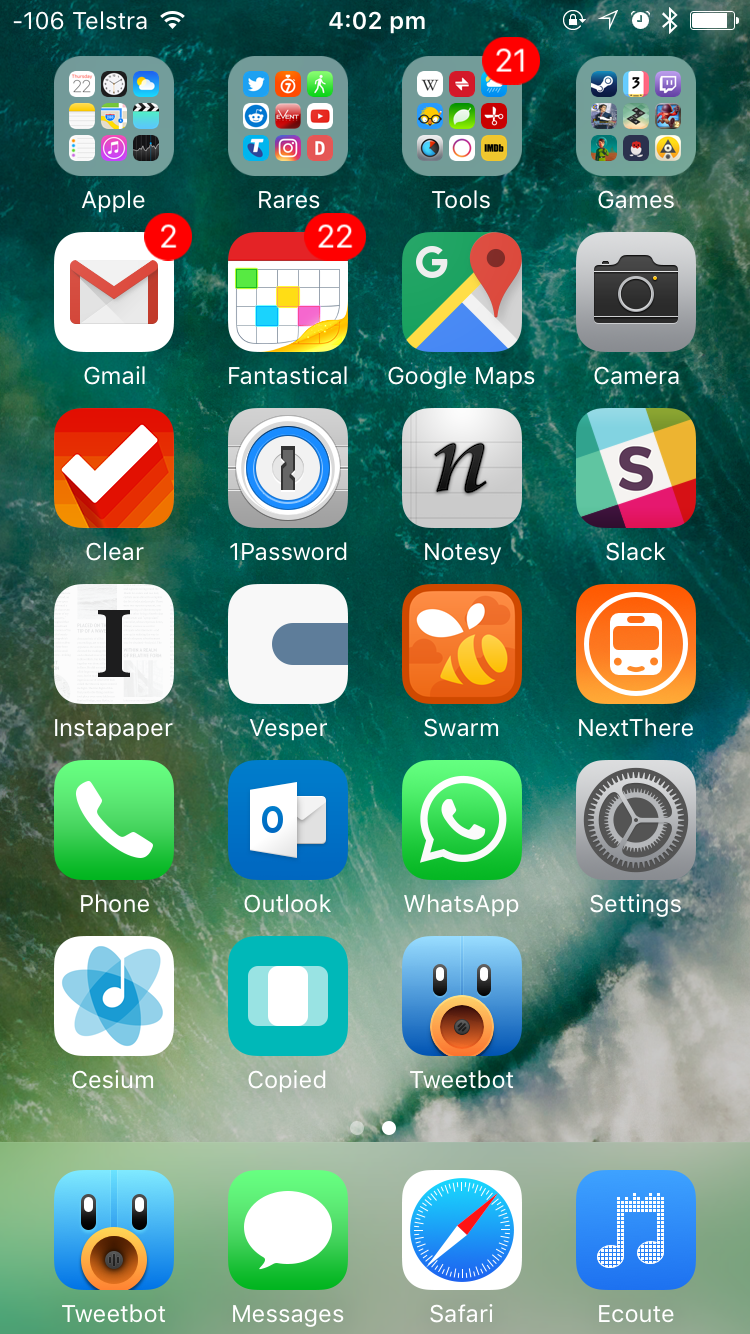A detailed screenshot of an iPhone running an older iOS version is displayed, showcasing a glimpse into a previous iPhone interface. The status bar at the top presents the time as 4:02 PM on the left side, alongside the Wi-Fi connection status, while the right side shows the battery level and various other standard icons.

The home screen layout comprises six rows and four columns of app icons, with a persistent dock at the bottom featuring four essential apps that remain static across all pages. Based on the presence of two indicator dots at the bottom, it is evident that there are two pages of apps, with the current screenshot displaying the second page as denoted by the highlighted dot on the right.

At the top of this page, the user has meticulously organized their apps into four folders labeled “Apple,” “Rares,” “Tools,” and “Games.” These folders encapsulate multiple apps, providing categorized storage and easy access. Below these folders, individual apps populate the screen, including Gmail, a password-saving app, Slack, and Tweetbot. Some apps are marked with red notification badges, indicating unread messages or pending notifications. The overall arrangement and design of the home screen reflect a structured and practical approach to app organization.